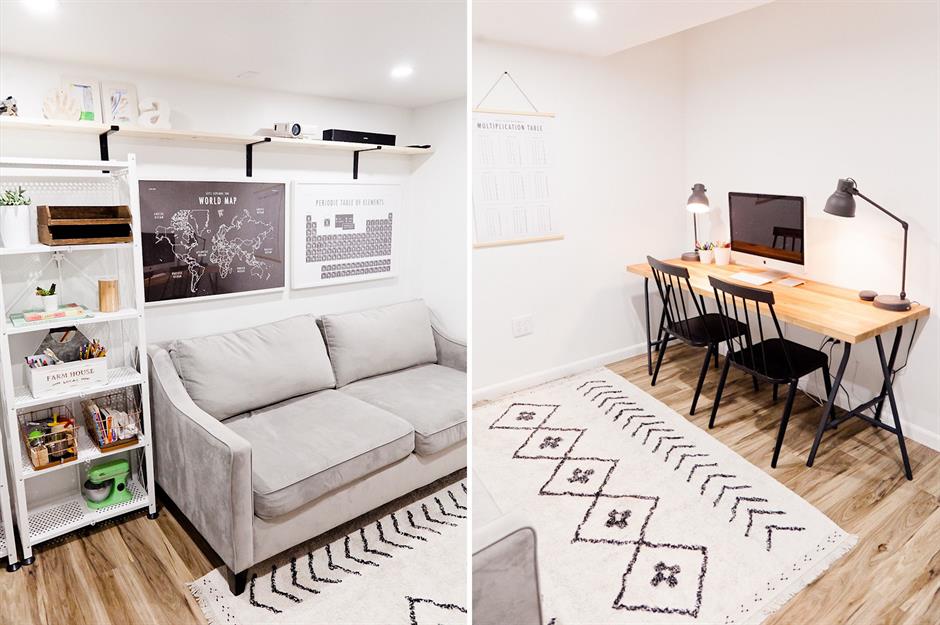The image depicts two sections of a living space in a side-by-side layout. On the left side, a light gray couch is centered against a white wall. Above the couch, there's a projector on a high shelf near the ceiling, and beneath it are two posters: a world map and a periodic table of elements. White multi-tiered standing shelves filled with various items such as candles, baskets, and crafts flank the scene. The floor in front of the couch features a black and white rug with a native pattern.

On the right side, the same black and white rug extends beneath a wooden desk that sits against the white wall. The desk supports a computer monitor and is flanked by two desk lamps on either side. Two black chairs are positioned under the desk, adding to the minimalistic style of the room. Subtle color tones of white, gray, black, light brown, and green unify the space, complementing the overall organized and cozy ambiance.